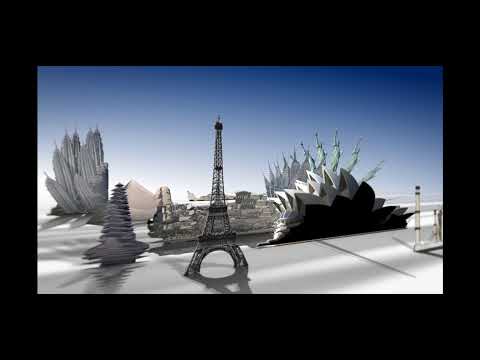The image is a detailed and somewhat grainy piece of computer-generated art showcasing a surreal composition of various iconic monuments. Dominating the center of the image is a tall replica of the Eiffel Tower. To the right, there is an intricate depiction of the Sydney Opera House, above which several overlapping Statues of Liberty fan out, creating a layered, almost animated effect. On the left side, there are ambiguous structures resembling cacti or stacked rocks, set in contrast to a distant pyramid-like shape, possibly the Great Pyramid, and remnants of what could be interpreted as the Great Wall of China. The scene is set against a muted, gradient blue-to-white sky, with the foreground depicted in silver or gray tones. The overall aesthetic is monochromatic and slightly blurry, lending an old-school, abstract feel to the 3D rendering.